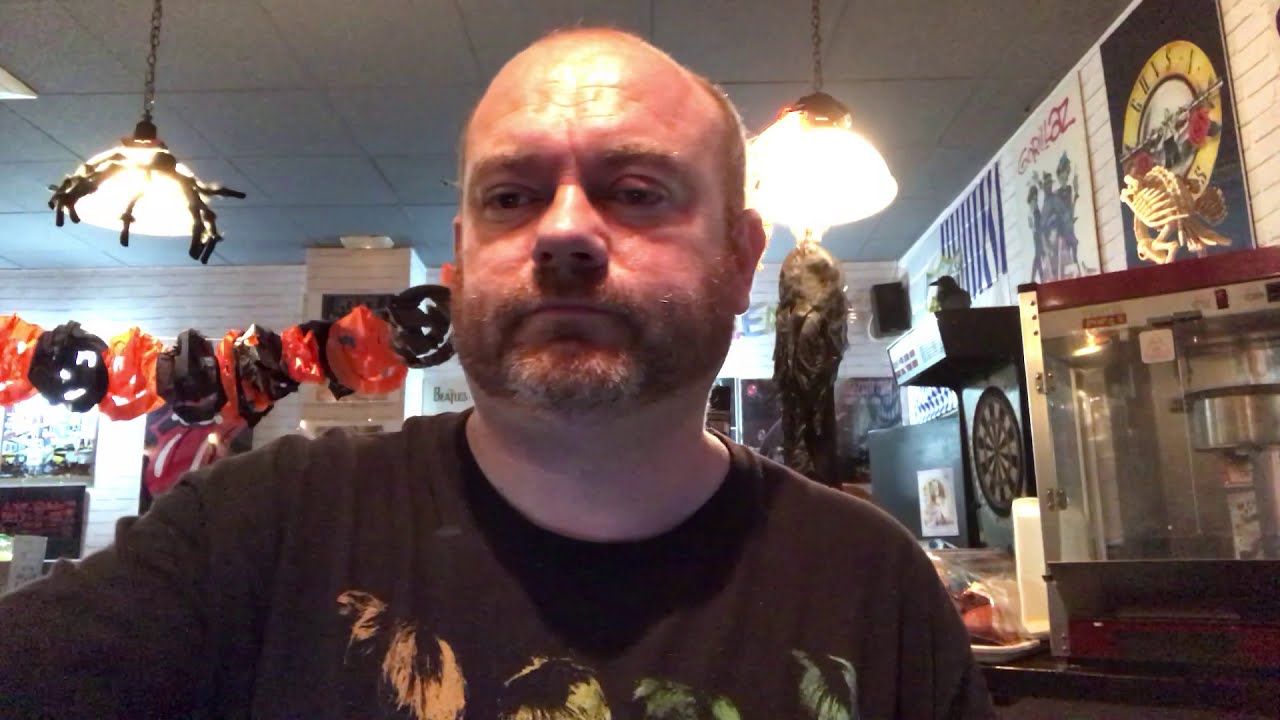The image features a man with a serious and slightly annoyed expression, occupying the left and center part of the frame. He has a round, reddish complexion, a bald top with some hair around the sides above his ears, and a trimmed strawberry blonde beard and mustache. His lips are tightly closed, giving him a grim look. The shine on his forehead is noticeable. He wears a dark shirt—either black or dark gray—adorned with images that are difficult to identify, though the top parts resemble four heads colored orange, yellow, green, and gray.

The background is set in a bar-like environment, decorated with rock and roll band posters and Halloween-themed items, including jack-o'-lantern paper cutouts strung from the ceiling. To the right of the man, there is a prominent Guns N' Roses logo featuring a gold circle and two pistols with roses. Additionally, there is a skeleton decoration atop what appears to be a popcorn machine. The setting includes two hanging lights, one on the upper left and another on the right side above the man's head.